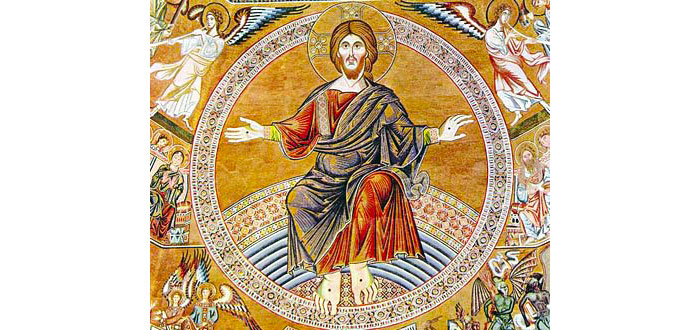This image portrays a detailed mosaic or mural featuring Christ at its center, encompassed by a near-edge white flowered circle. Christ, identifiable by the halo around his head, sits with his hands extended to his sides, palms up, both with holes in the center. Notably, his left hand is depicted upside down. He wears a long red robe beneath dark brown robes, complemented by a bluish, purplish, yellowish sash. Christ's feet are bare, with visible holes, and he has long brown hair and a full beard.

Surrounding Christ, the background transitions from dark to light brown. The upper corners of the image showcase angels playing harps or trumpets, while the bottom corners contain darker figures and additional winged entities. To the left and right of Christ are people clad in similar robes; these figures also feature halos, indicating their saintly status. These intricate details contribute to the overall sacred and complex depiction.